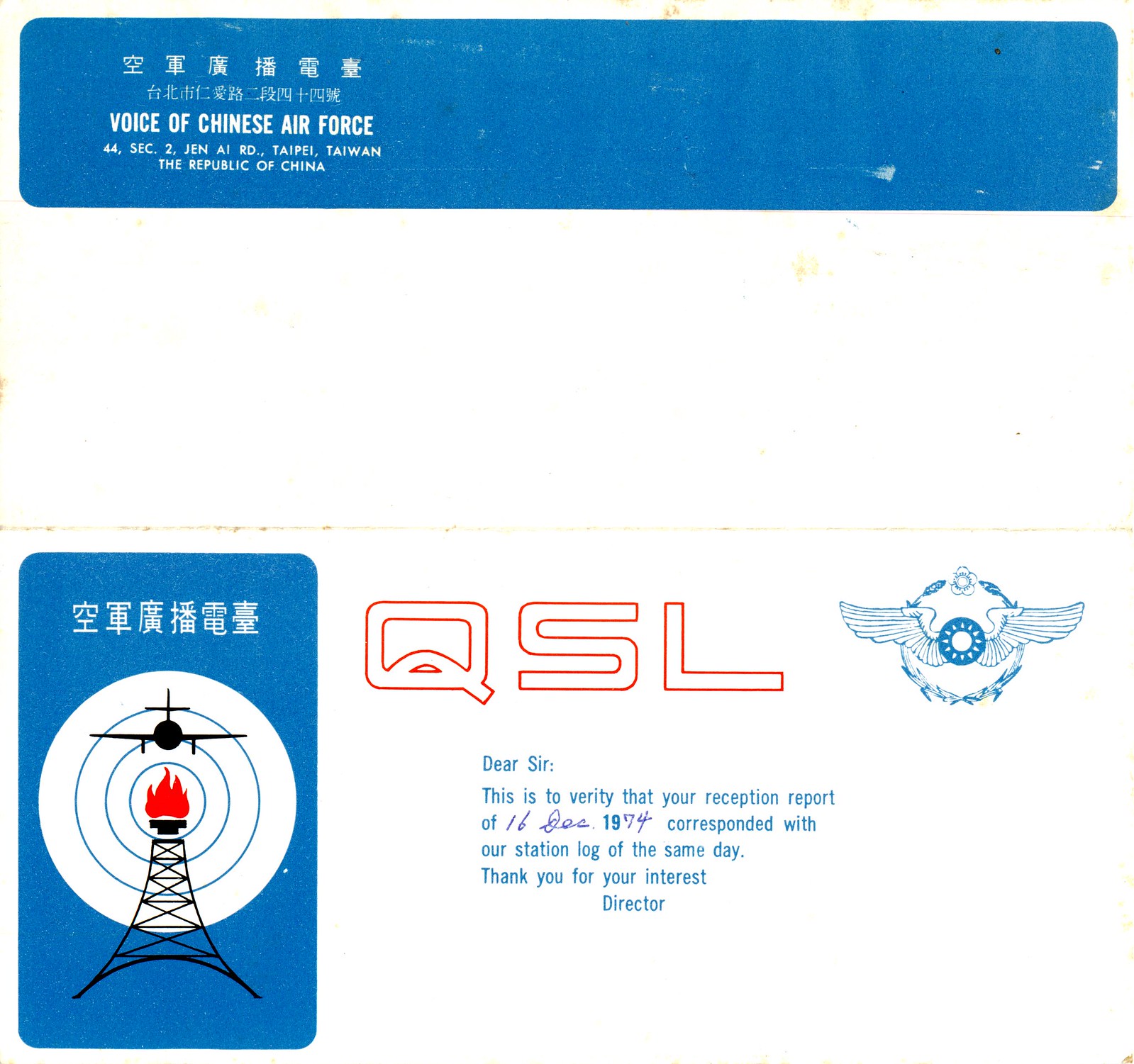The image is a postcard from China, titled "Voice of Chinese Air Force," originating from Taipei, Taiwan, Republic of China. It features a distinct design divided into two main sections, both set against a white background, marred by some yellow spotting and staining. 

The top half of the postcard has a deep blue banner at the top, with white text including Chinese characters and the lines, "Voice of Chinese Air Force, 44, SEC.2, GEN AIRD, Taipei, Taiwan, Republic of China." Below this banner, the section remains blank.

The bottom half of the postcard is more intricate, dominated by a vertical blue rectangle on the left side. The top of this rectangle displays more Chinese text in white. Beneath the text is a white bullseye or darts target with blue details. At the top of the target is a black airplane silhouette with a red fire symbol beneath it. Further down, there's an image resembling a black radio tower or oil derrick.

In the middle-right of the bottom half, the large red-bordered letters "QSL" stand out, followed by a verification note in blue text: "DEAR SIR: This is to verify that your reception report of 16 December 1974 corresponded with our station log of the same day. Thank you for your interest, Director."

To the top-right of this bottom section is a blue-outlined logo featuring a circular wreath with a central sun-like design and wings extending on either side, adding a distinctive touch to the postcard’s official verification theme.